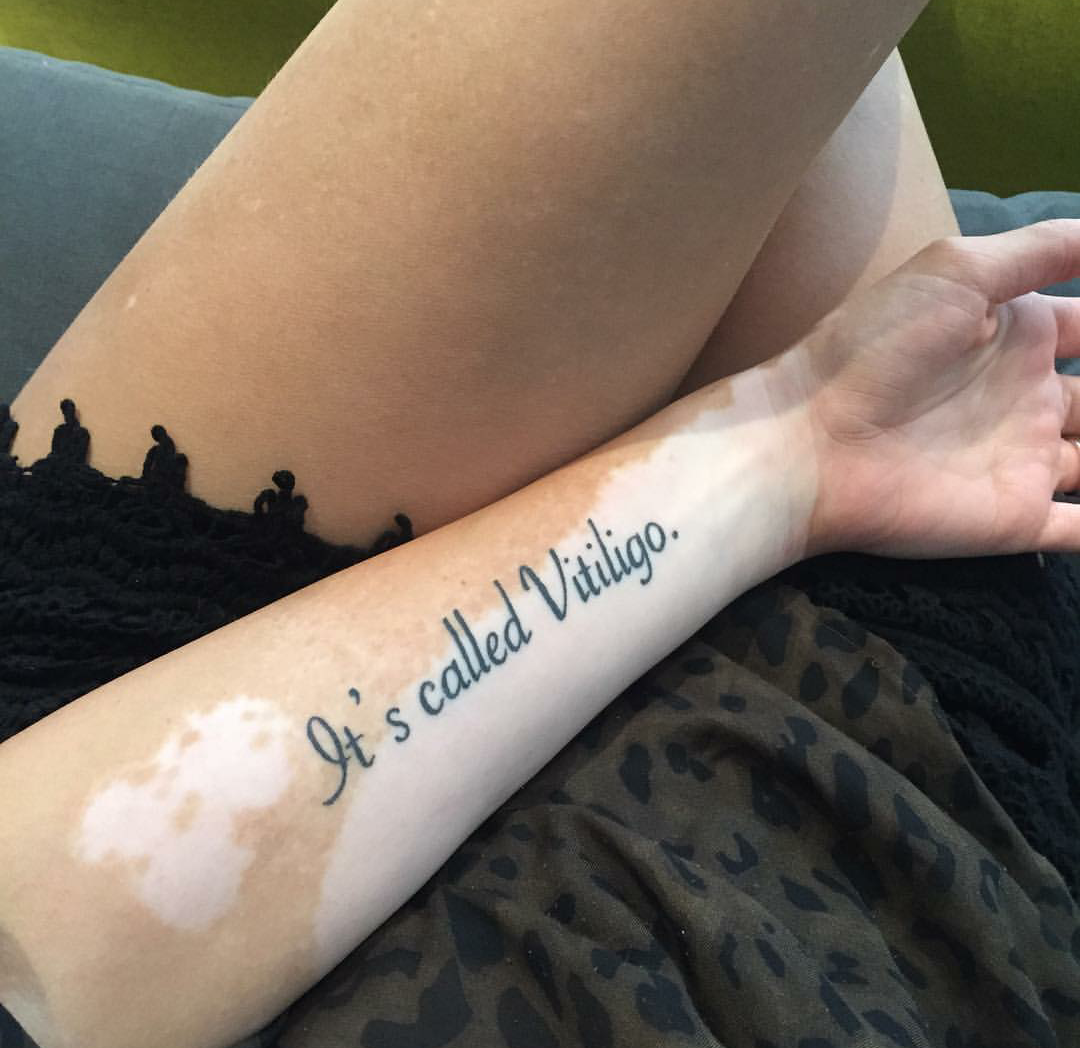The image captures a close-up of a person's crossed legs and their inner forearm, prominently featuring a tattoo that reads "it's called vitiligo" in black letters. The individual's skin shows distinct patches of vitiligo, where areas of their natural light tan complexion turn white. The person appears to be seated on a blue couch, wearing black, frilly shorts, and a greenish-black leopard-print top. There is a clear contrast between the bright whiteness of the vitiligo patches and the rest of their light brown skin. The setting is brightly lit with natural light, emphasizing the tattoo and the texture variations of the skin. The entire scene exudes a personal and candid feel, suggesting that the photo might have been taken by the individual themselves to capture and share their unique skin condition deliberately.